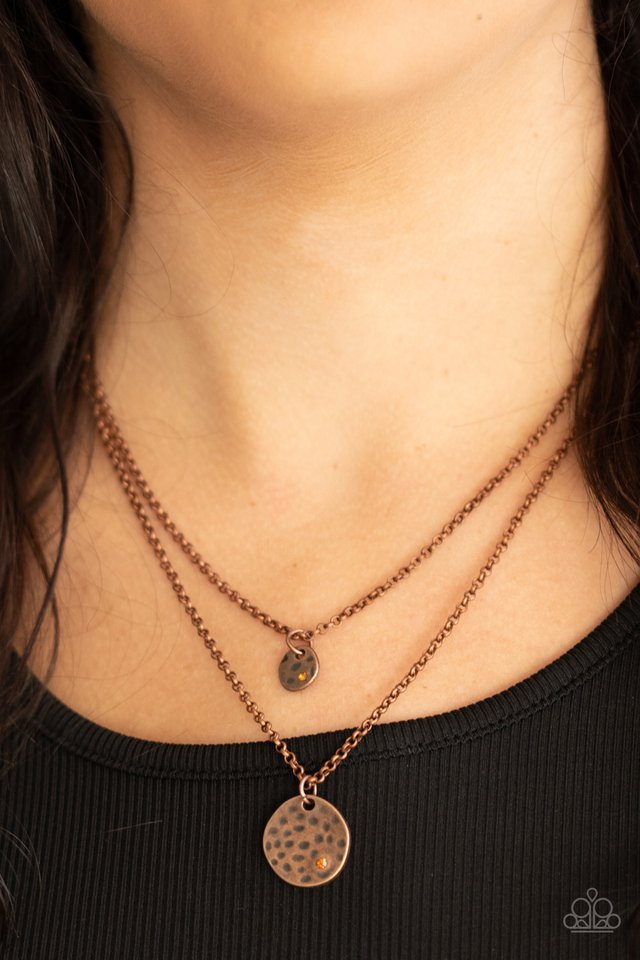This close-up photograph captures a detailed view of a woman's neck adorned with two distinct necklaces, showcasing her long, dark brown wavy hair and fair skin, which suggests she could be Caucasian or possibly Latina. The frame extends from her chin down to just beneath her collarbones, emphasizing the jewelry against her black ribbed shirt.

The necklaces, slightly tarnished, appear to be made of copper or a similar bronze-like metal. The upper necklace features a smaller circular pendant, while the lower necklace displays a larger pendant, both with hammered textures and gray indentations, giving them a handmade look. The larger pendant on the bottom additionally seems to have a small gemstone at its base. The fine details of the necklace chains and pendants are key highlights of the image. In the lower right corner, there is a white watermark logo resembling a pyramid of stacked circles with a floating upside-down teardrop shape above, suggestive of a stylized crown.